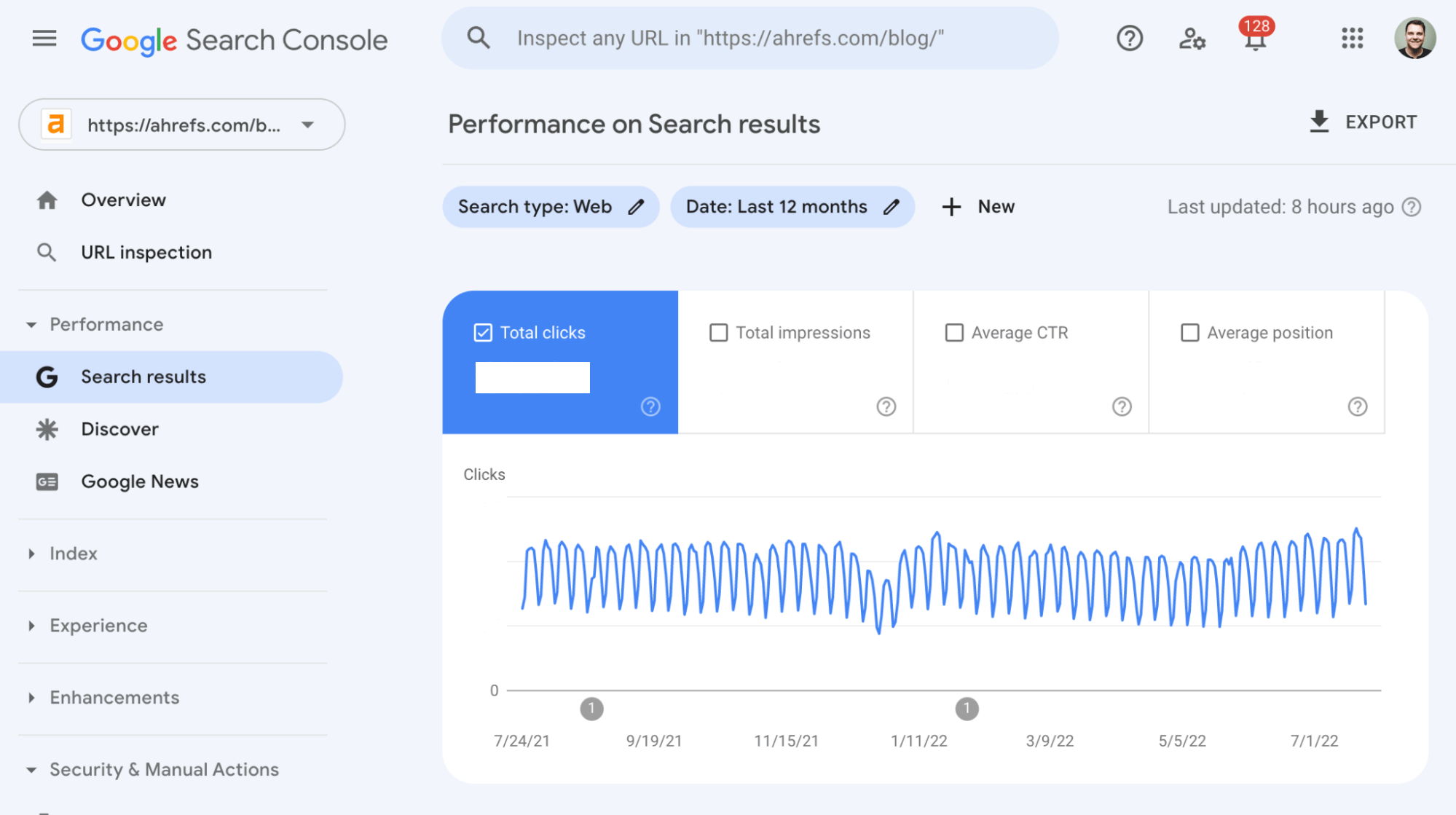The image is a rectangular screenshot of the Google Search Console interface set against a very light blue background. At the top left corner, the word "Google" is prominently displayed in its iconic colorful letters, featuring blue, red, yellow, and green. Right next to it, "Search Console" is written in gray. To the right of the title is a search bar with the placeholder text "Inspect any URL in https://ahrefs.com/blog."

Adjacent to the search bar is a help icon represented by a question mark inside a circle. Following the help icon are a series of icons: a user profile icon, a notification bell marked with a red indicator showing 128 notifications, an all-apps grid icon, and a profile photo of a smiling man.

Below the header, the text "Performance on Search Results" is displayed in black. Underneath this title, there are two filter buttons labeled "Search Type: Web" and "Date: Last 12 Months," accompanied by text indicating that the data was last updated 8 hours ago. There's also a "+ New" option for adding new elements.

Further down, several tabs are available for selection: "Total Clicks," "Total Impressions," "Average CTR," and "Average Position." The section below these tabs features a graph displaying performance data, where a bright blue, squiggly line charts the data points from left to right.